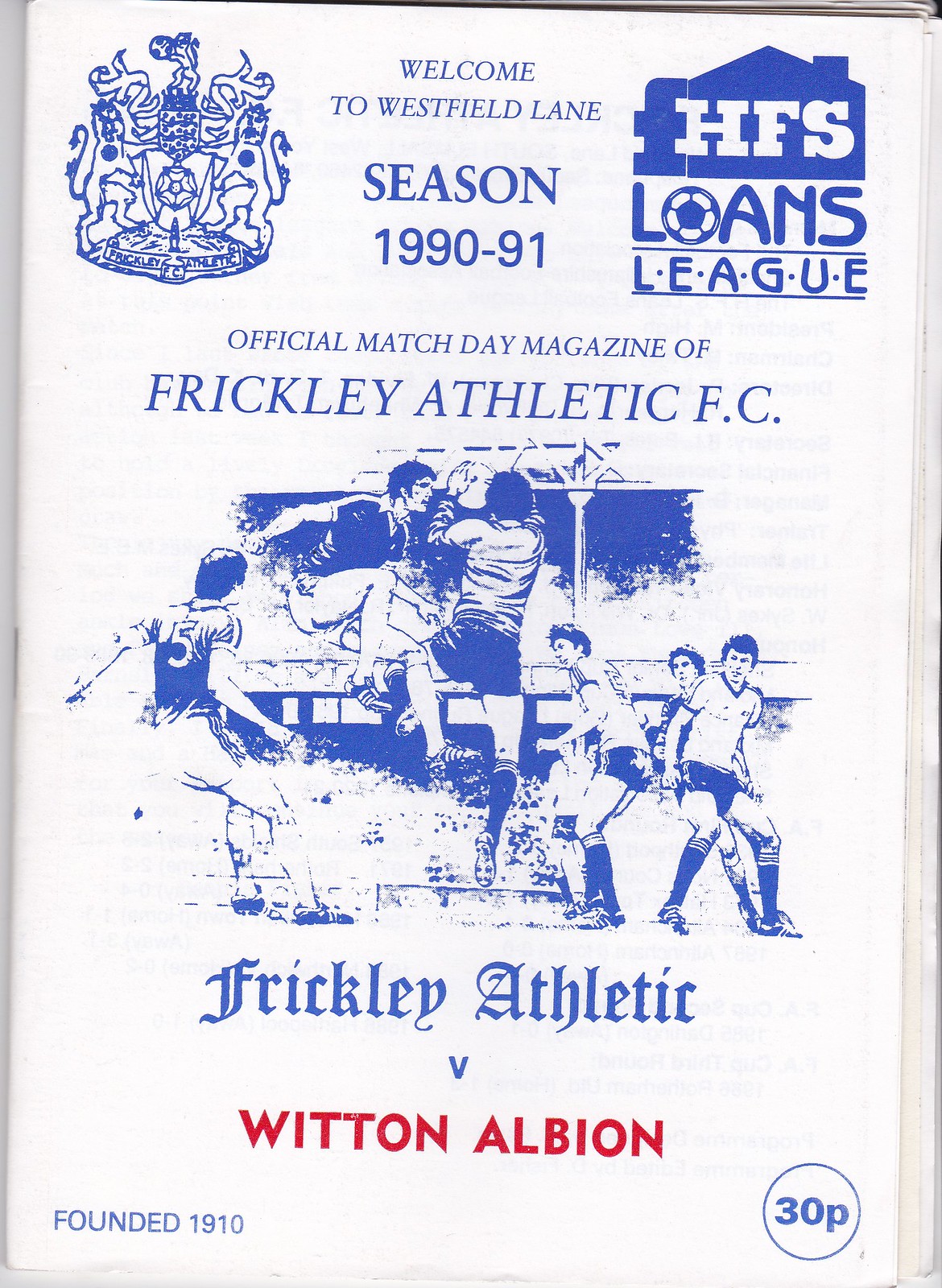This detailed descriptive caption combines the key elements and shared details from each voice caption:

The image is the front page of a match day magazine for Frickley Athletic FC titled "Welcome to Westfield Lane, Season 1990-91, Official Match Day Magazine of Frickley Athletic FC." The page features a blue and white illustration of a rugby match, though the players are dressed in traditional soccer attire, including cleats and shorts. There are six boys in total, with two in the center of the image jumping high, one on the right holding a soccer ball, and another trying to intercept it. The boys are wearing different colored uniforms: those in white shirts have blue shorts, and those in blue shirts have white shorts. The illustration is set against a backdrop that suggests a full stadium, enhancing the sense of action and competition.

The top left corner of the page displays the Frickley Athletic FC emblem, featuring two heraldic griffins or lions holding a shield. In the upper right corner, there's an icon of a house with the text "HFS Loans League." At the bottom of the page, it reads "Frickley Athletic vs. Witten Albion," with "Founded in 1910" on the bottom left and "30p" in a blue script inside a circle on the bottom right, indicating the price of the program. Overall, the design and details reflect the official nature of the match day magazine for the 1990-91 season.